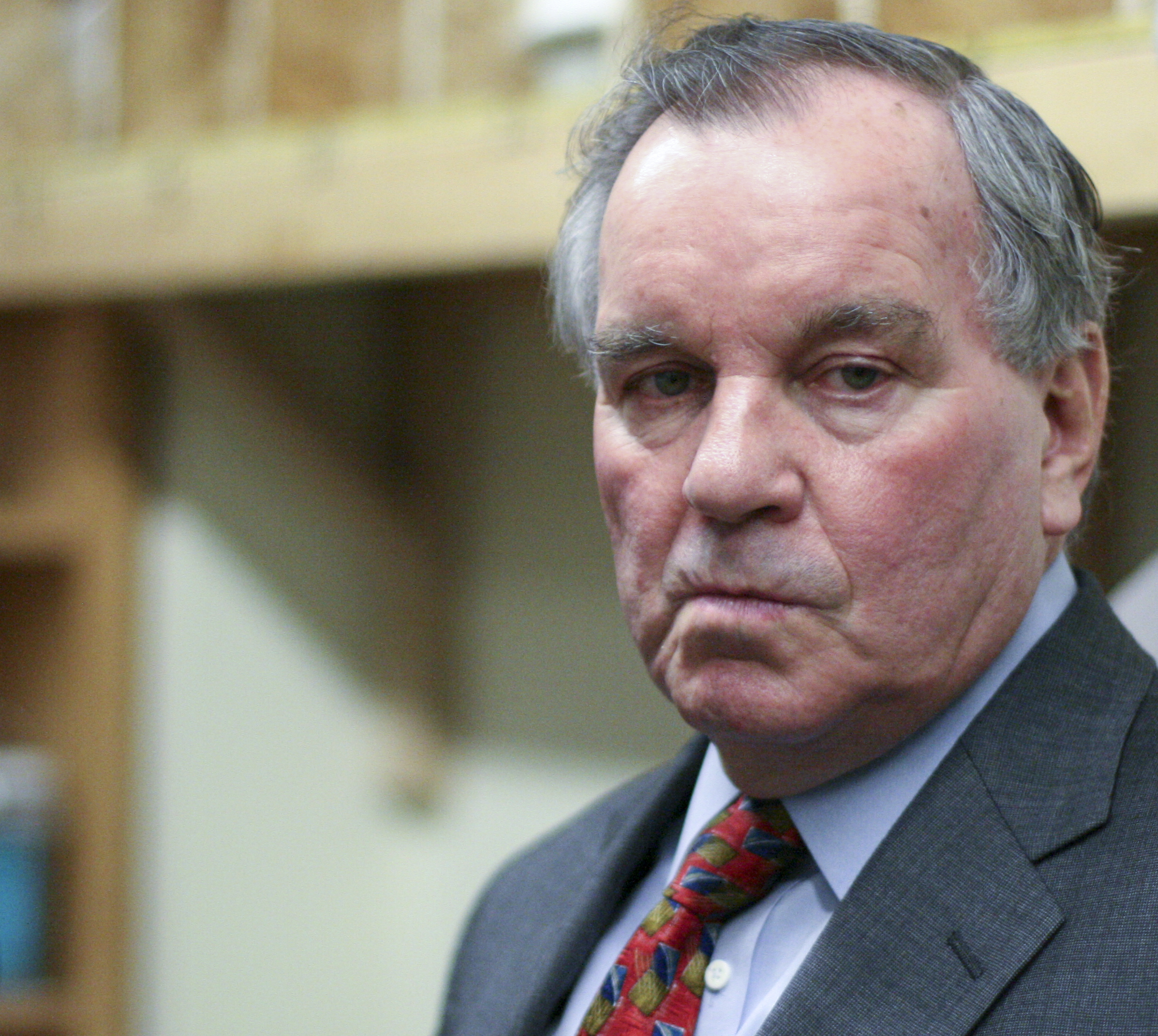This image depicts a stern-looking older man, likely a politician or businessman, in his late 60s or early 70s. He is dressed formally in a dark gray tweed suit jacket over a light blue, almost white, button-down collared shirt, paired with a red tie featuring blue and yellowish squares. His hair is short, predominantly gray with remnants of brown, and slightly unkempt, extending over his ears. His highly receding hairline reveals a high forehead, and he has salt-and-pepper gray eyebrows. His face is craggy with visible wrinkles, jowls under his chin, and a tightly pressed mouth. The man's eyes are dark, though their exact color is not distinguishable in the photograph. He is positioned mostly on the right side of the image, facing three-quarters to the left but looking directly into the camera. The background is blurred, showing a room with white or light green walls, wooden trim, and possibly a two-story structure with a balcony or wooden railing. The left side of the image hints at either a door or wooden shelving.